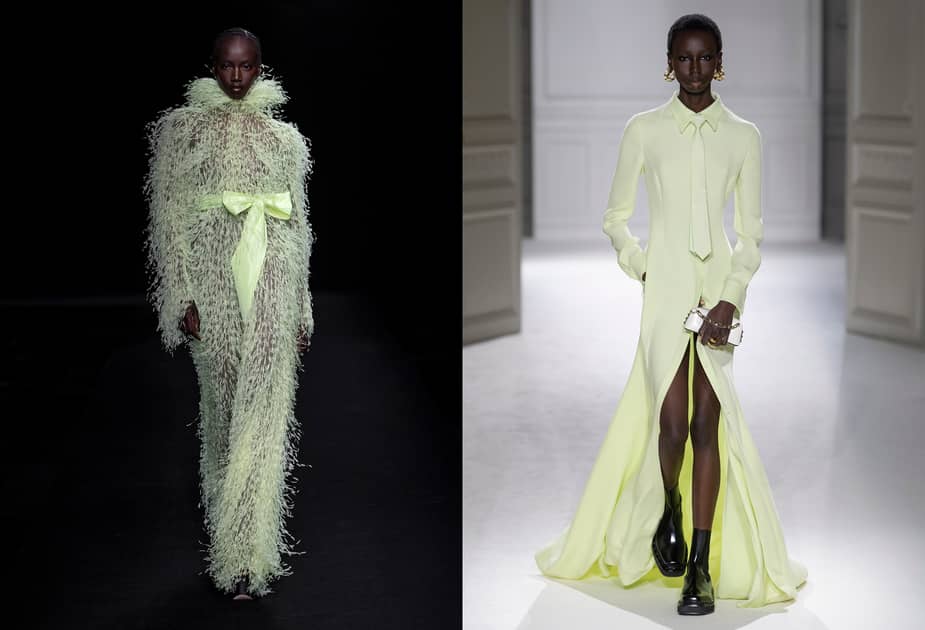In this side-by-side photograph, we see a striking model with very dark brown skin and closely cropped, textured hair, showing off two distinctive outfits. The left image features her against a black background on a runway, emphasizing an avant-garde, high-fashion ensemble. She's adorned in a long-sleeved, yellow mesh dress with a high collar and a silk ribbon cinching the waist, revealing her skin beneath. The material gives off a fur-like, almost plastic-textured appearance from a distance, creating a dramatic, eye-catching effect. 

In contrast, the right picture showcases the same model in a more structured setting with off-white and white wooden molding and white flooring. Here, she poses in a light yellow, long-sleeved dress with an oxford collar. This dress features a bold central slit reaching up to her mid-thigh, accentuated by a tie around the belly button. She completes this chic look with black, shiny anklet boots and a white clutch in hand, paired with delicate earrings. This captivating juxtaposition highlights both the versatility of the model and the creativity of the fashion.